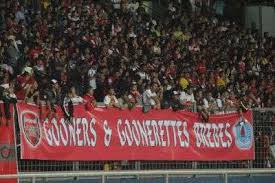The image depicts a crowded stadium with bleacher-style seating, filled with an enthusiastic audience. At the forefront, a red rectangular banner is draped over a railing to prevent spectators from falling. The banner prominently features the words "Gooners and Goonerettes" in uppercase white letters. The writing extends to another word, "BREBES," though partially obscured by wrinkles and the photo’s lack of focus. On the far left of the banner is a red shield emblem, while a blue logo is displayed on the far right. The dense crowd, packed tightly in the stands, suggests the scene is from a sporting event, though the actual field of play is not visible in the photograph.